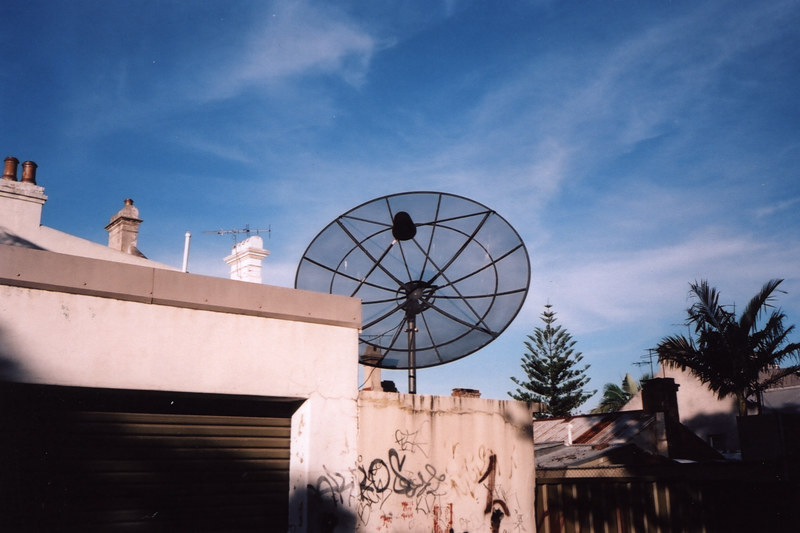The photograph features a slightly grainy, vintage image of a black and gray, see-through mesh satellite dish centered atop a cream-white building with a brown garage door. The foreground to the left shows another garage with a brown door, part of an off-white structure adorned with graffiti, mostly black with some red. The notable graffiti letters "R-O-S" and an "L" are visible. To the right of the main building, partly obscured by shadows, stands an old wooden house or possibly another garage. Bright sunlight illuminates the scene, suggesting a tropical location, with a tall palm tree on the right. Above the satellite dish, the sky is bright blue with scattered cirrus clouds. Additionally, to the middle right, there are rooftops with chimneys and possibly TV antennas, which add to the urban landscape.